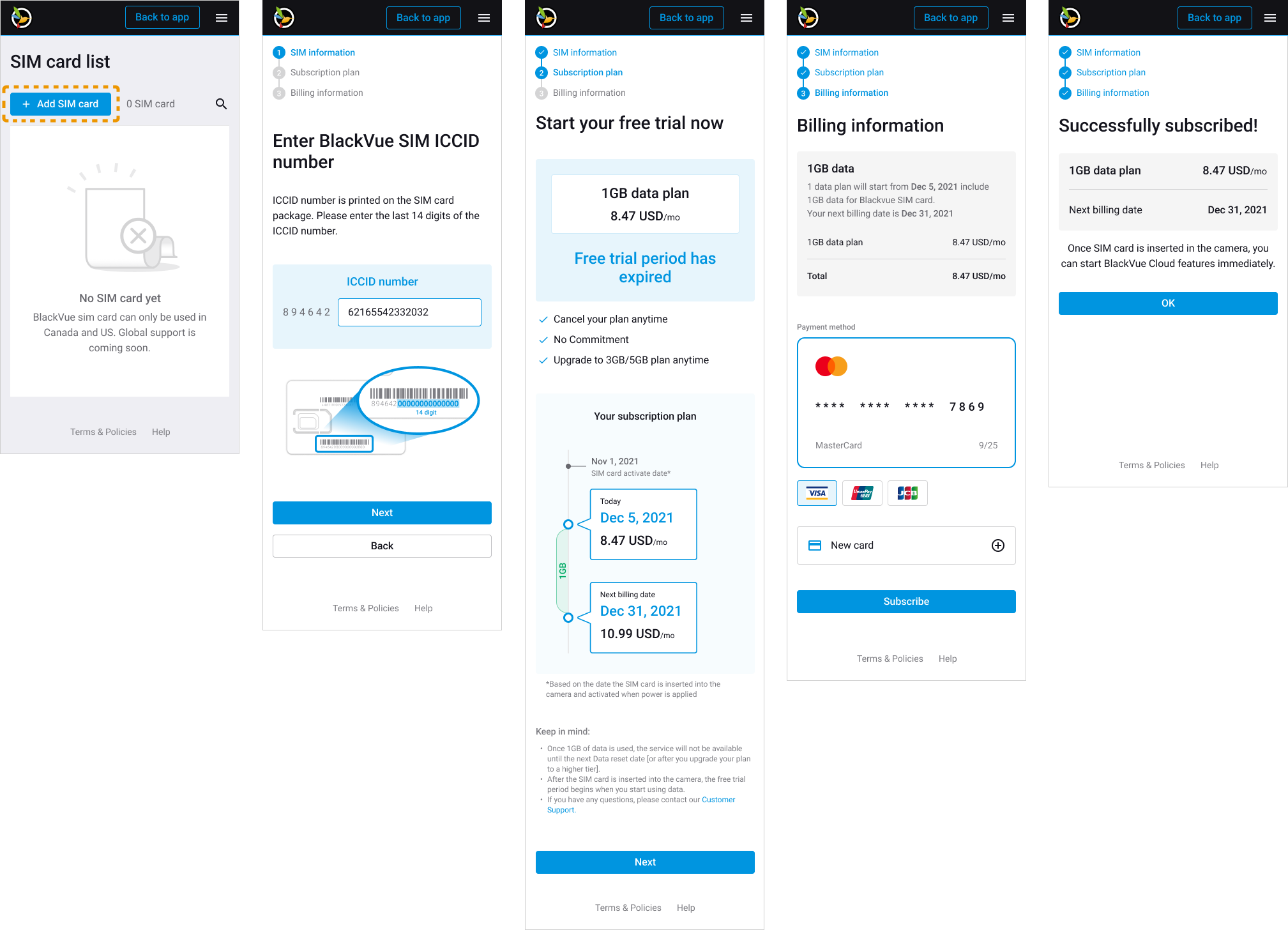A series of five screen captures from a mobile device, each varying in length and height, detailing a SIM card setup process. At the top of each screen, there's a black bar with a hamburger menu on the right and a logo on the left. 

1. The first screen displays the title "SIM Card List" with an "Add SIM Card" button outlined in orange. Below it, there is a grayed-out message stating "No SIM card yet."

2. The second screen is a prompt to "Enter BlackVue SIM ICC ID Number," with a numerical entry field and "Next" and "Back" buttons below it.

3. The third screen is titled "Start Your Free Trial Now" describing a 1GB data plan priced at $8.47 per month. It mentions that the free trial period has expired with the subscription plan initiated on November 1, 2021. The current date is December 5, 2021, with the next billing date set for December 31, 2021.